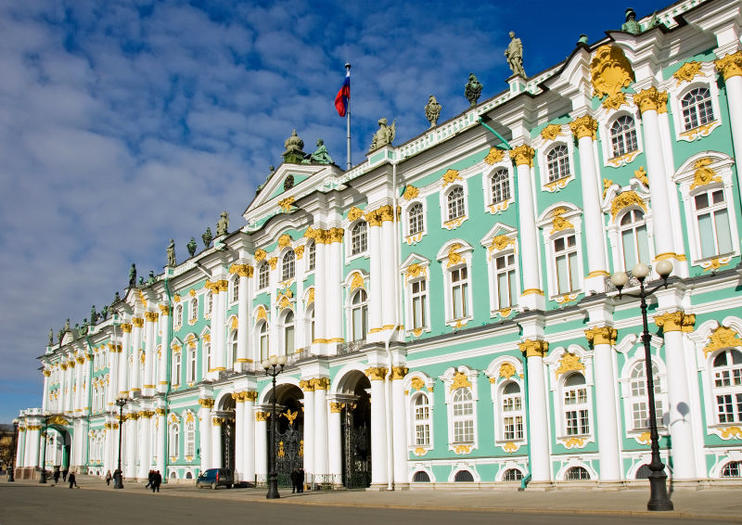This image showcases a grand and historic building complex with a striking facade of white and mint green, adorned with intricate golden etchings. The structure features multiple stories, likely three or four, and is embellished with numerous closely set windows and columns that stretch from the ground to the roofline. The entrance is marked by three arched doorways surrounded by white columns. Topping the edifice are twenty to thirty statues depicting various figures and animals, lining the roof's entire length. The building is set against a backdrop of a blue sky dotted with gray and white clouds. At ground level, there is an asphalt road and a gray concrete sidewalk edged in yellow, punctuated by black metal light poles each adorned with three globe lights. People are seen walking around the premises, adding life to the scene, while a flag bearing red, blue, and possibly white colors flutters atop a flagpole, ambiguous in its national association. The overall architecture suggests an opulent, possibly royal or governmental building, exuding an air of historical grandeur.